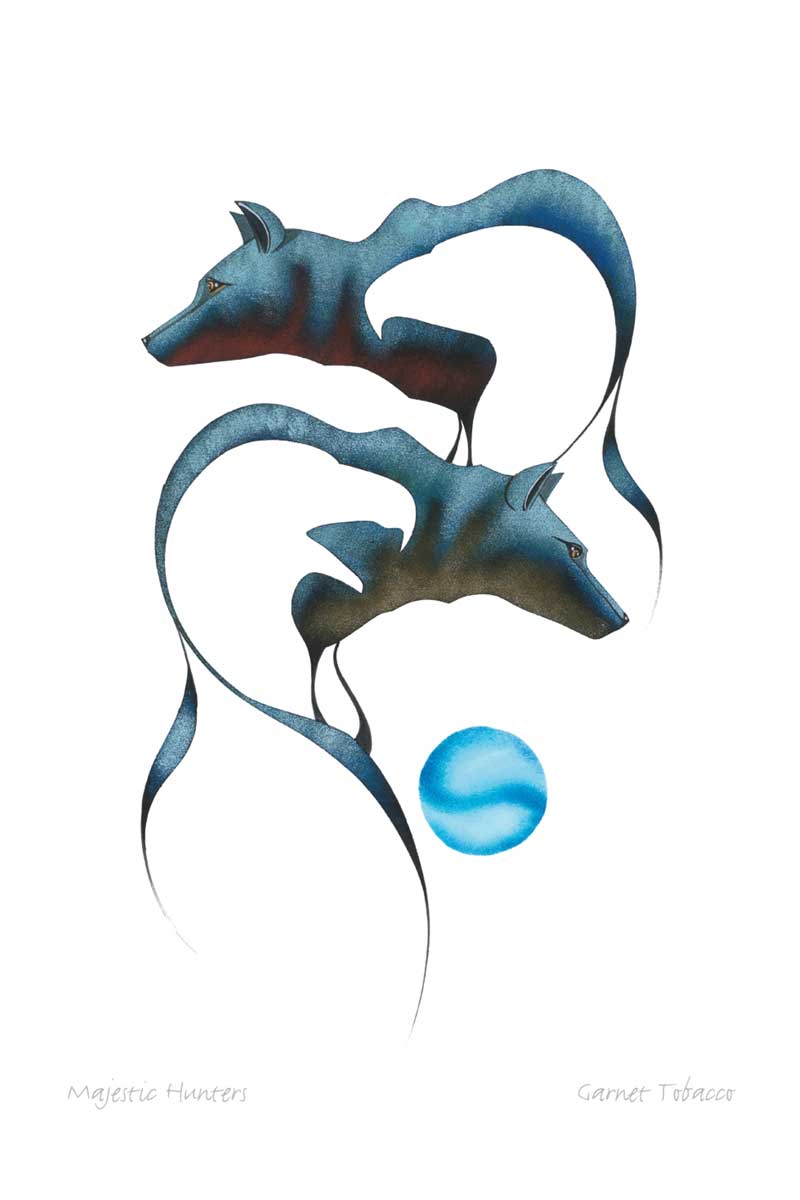The image depicts a detailed and intricate illustration set against an all-white background. It showcases two wolves, one positioned on top of the other. The top wolf, tinged in bluish-gray, faces to the left, while the bottom wolf, shaded similarly, faces to the right. Both wolves exhibit hollowed-out bodies, filled with negative space that creatively forms the silhouettes of birds. The bird within the top wolf has its beak closed and curves downward, while the bird in the bottom wolf has an open beak, also curved downward. Beneath the bottom wolf, there is an orb of swirling navy and light blue hues, resembling a marble or moon. The text "Majestic Hunters" is displayed in the bottom left corner, and "Garnet Tobacco" is faintly inscribed in gray on the bottom right.